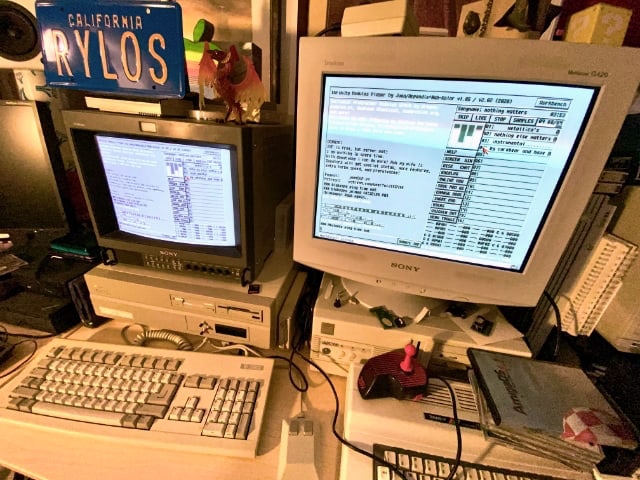The photograph captures an indoor computer room with a horizontal rectangular layout, featuring two older model Sony computers on a light-colored desk. In the upper left corner of the image, a dark blue California license plate with light brown text reads "R-Y-L-O-S." Below the license plate, there is a dark gray, boxy CRT monitor atop a computer tower. The screen displays a blue background with some charts, while a beige keyboard sits directly in front of it. Adjacent to this is another older style, white CRT monitor placed higher up on another computer tower, also showing a blue background with charts. This setup includes a white keyboard and a small joystick with a black cord resting on the desk. Further to the right, behind the second monitor, are shelves cluttered with various objects, including CD cases and notebooks. Nestled to the right of the license plate is a small, red plastic figurine resembling a pterodactyl, adding a unique touch to the nostalgic tech-centric scene.